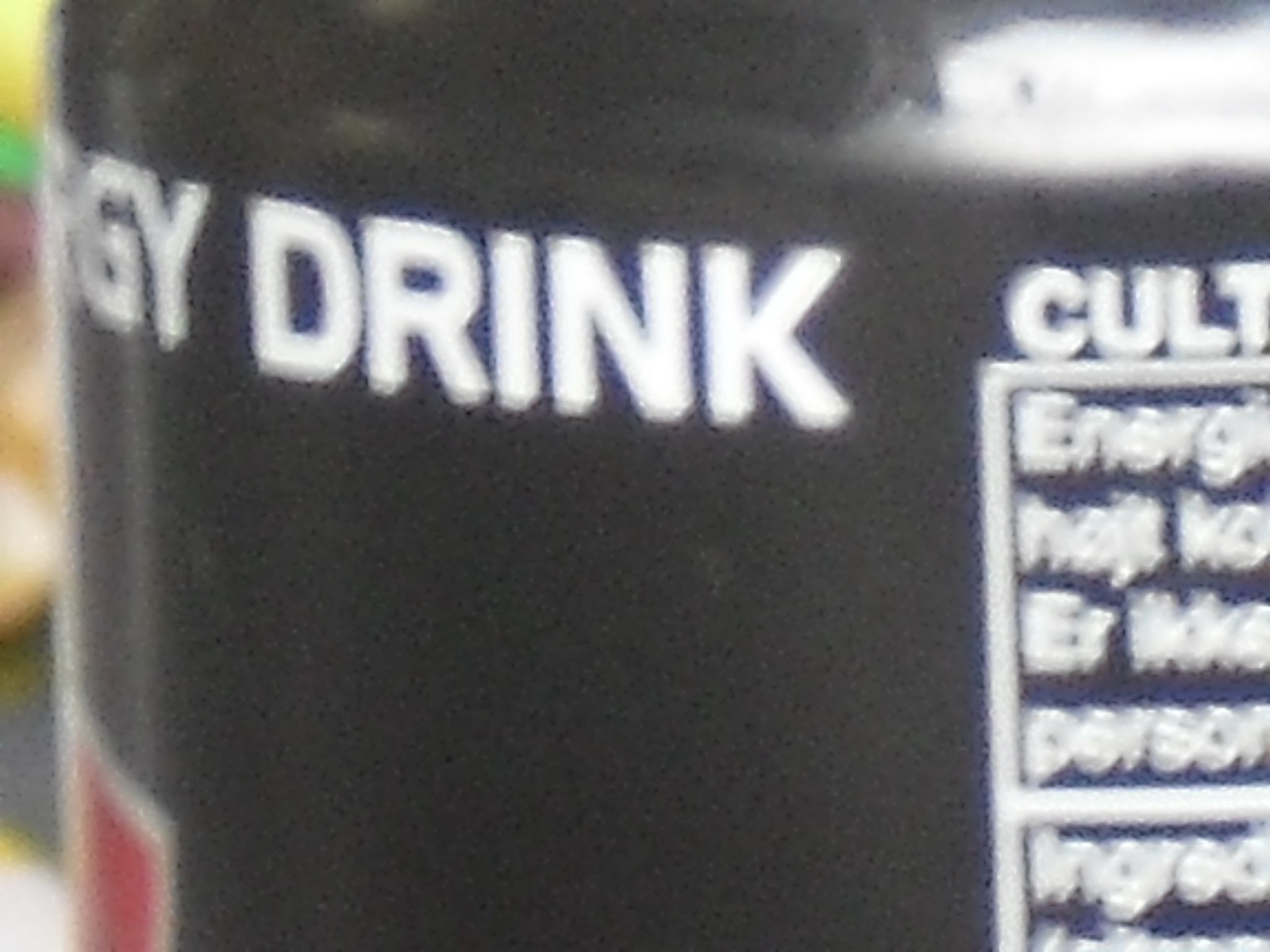A blurry photograph captures a partial view of a black can with red accents on its label. The can is an energy drink, but only fragmented letters "G Y D R I N K" are visible, obscuring the full word "energy." The image also includes a portion of the nutrition label in the lower right-hand corner. Prominently displayed on the can are the letters "C U L T" in white, set against a white box featuring the word "energy," followed by two illegible lines, then the word "person," another line, and finally the word "ingredients."